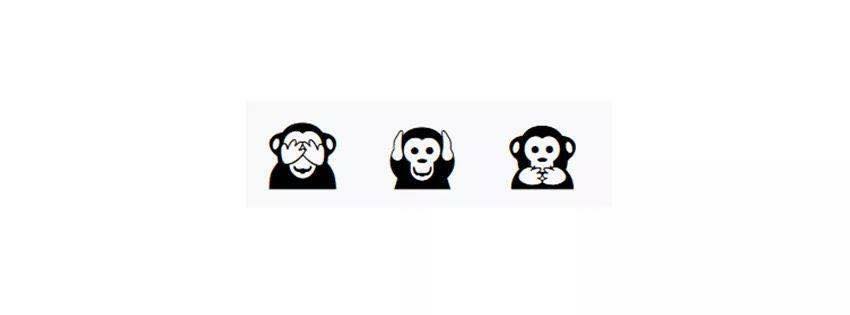This is a very small, low-resolution photograph of a rectangular strip of fabric or paper with a slightly darker white or gray outline than its white background, heavily pixelated with visible JPEG artifacts. The fabric features three simple black and white illustrations of monkeys performing the "see no evil, hear no evil, speak no evil" gestures. Each monkey has a black body with white faces, hands, and inner ears.

The monkey on the far left covers its eyes with its hands, displaying a smile beneath the hands. The middle monkey covers its ears, showing black circles for eyes and an oblong shape for the nose, all against a white face, and also wears a smile. The rightmost monkey, identical in coloration, covers its mouth with its hands. All three monkeys are evenly spaced along the fabric strip, contributing to a consistent and harmonious design. The simple, black-and-white graphical style highlights the classic moral adage these monkeys represent.